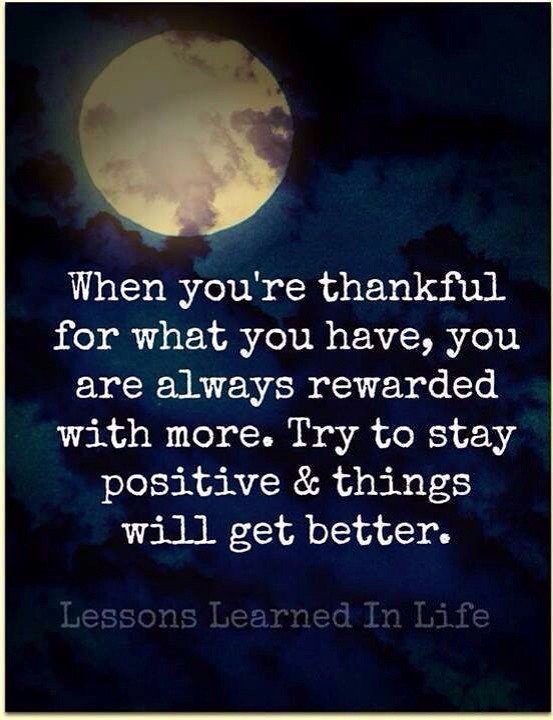The image is a vertically aligned rectangle with a predominantly dark blue and black background, depicting a night sky. The upper left-hand side features a bright yellow full moon partially covered by clouds, which appear to be a mix of black and purple shades, flowing from right to left. Centered below the moon is a motivational quote in white text: "When you're thankful for what you have, you are always rewarded with more. Try to stay positive and things will get better." At the bottom of the image, there is additional text in gray that reads "lessons learned in life," also centered. The overall composition of the image suggests an inspirational meme, potentially suitable for framing or sharing on social media.